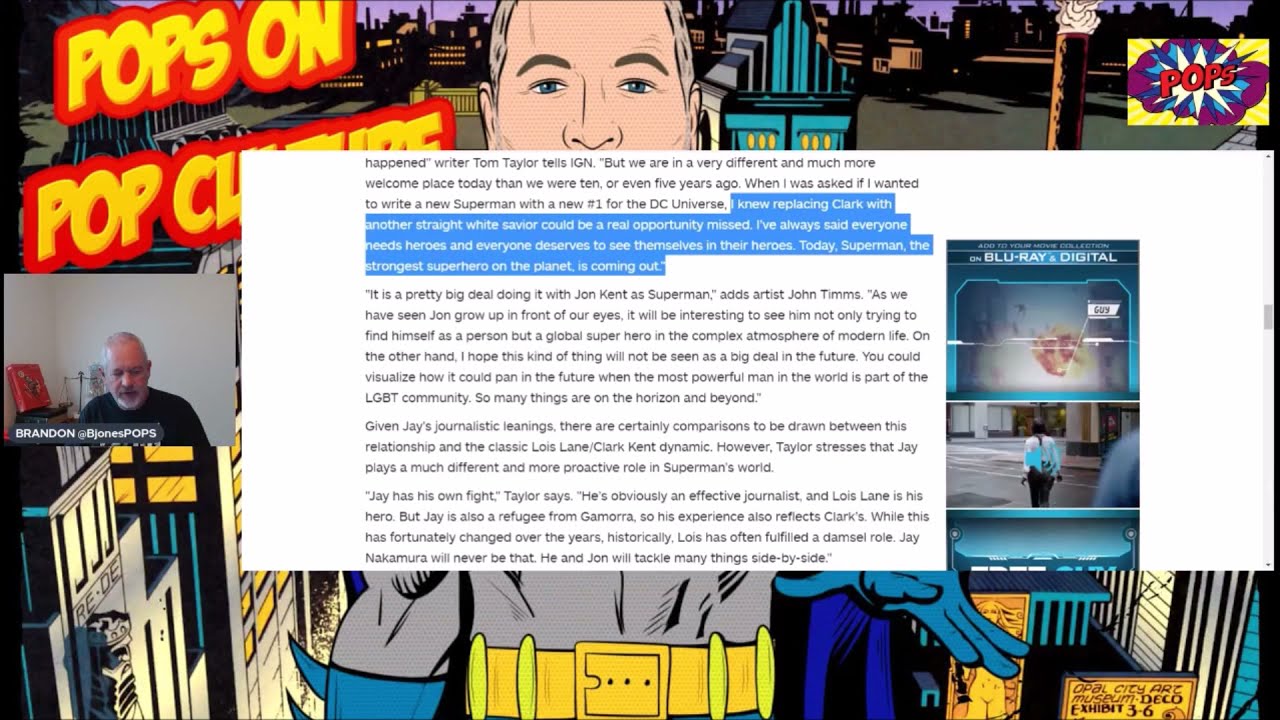The image is a horizontal rectangular comic strip style, predominantly animated, with various textual and graphical elements. In the upper left-hand corner, large yellow letters outlined in red spell out "POPS," with the partly obscured words "on Pop Culture" beneath them. A central section features an animated superhero in a gray uniform with blue gloves and a gold belt, though only his blue eyes, gray hair, and the upper portion of his head are clearly visible as a large white text box filled with paragraphs covers the rest of his face down to his chest. This text seems to comment on cultural representation in superheroes, highlighting phrases like, "I knew replacing Clark with another straight white Savior could be a real opportunity missed" and "everyone needs heroes and everyone deserves to see themselves in their hero. Today's Superman... is coming out."

Adjacent to this, the right side of the image displays a small square section with a gray wall background, showing a human character—a man with short gray hair, beard, and mustache—identified as "Brandon" in all caps white letters, followed by "at B. Jones pops." In the upper right-hand corner, a small, colorful rectangle contains red letters spelling "POPS," surrounded by white, blue, purple, and yellow backgrounds.

In summary, the image also features a podcast or streaming element. On the left, there is a window showing a streamer, a man with gray short hair and a gray beard, wearing a black t-shirt. He appears to be watching content, possibly a web browser displaying a video or text content. Overall, the backdrop seems custom designed to match the branding of a channel titled "Pops on Pop Culture."